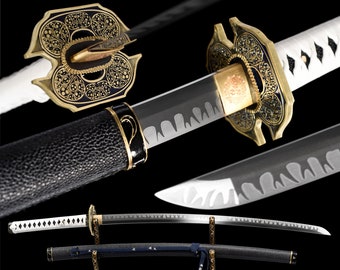This image displays a compelling arrangement of four elaborate oriental swords, including a distinct Japanese-style sword, all starkly set against a jet-black background in a landscape format. At the very bottom, a full-length sword is showcased with its black arced sheath, adorned with bronze elements at both ends. Above this, a detailed view of the sword reveals a white handle featuring a single row of black diamonds, a golden handguard, and a slightly curved silver blade. Higher up to the right, the sharp tip of the blade is visible, exhibiting a wavy pattern in lighter grey along its edge. Moving further up, another sword is depicted partially unsheathed, with its black sheath on the left and the blade extending several inches outward. Finally, at the top, a close-up perspective highlights the very tip of a sword pointing upwards, focusing on the face of its golden handguard. This intricately detailed image seems like a professional display, potentially for advertisement purposes, to showcase the craftsmanship and design of these exquisite swords.